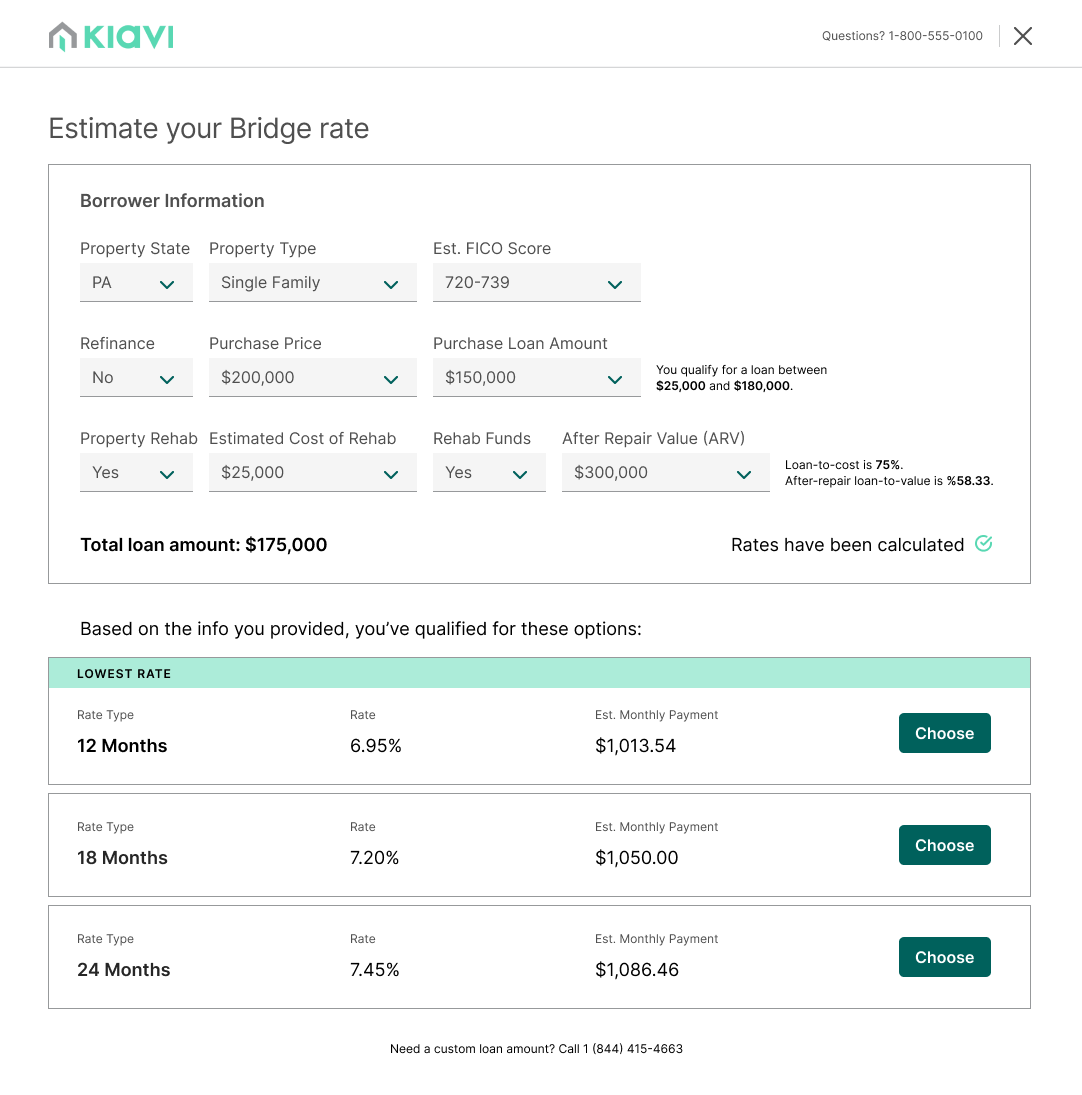### Detailed Caption for the Financial Information Screenshot

The screenshot depicts a webpage from KIAVI focused on financial information and estimating bridge rates, with a predominantly white background. 

**Header Section**:
- **Top Left**: Features the KIAVI logo, which includes a grey outline of a house containing a teal green shape resembling a rhombus or diamond. To the right of the logo, "KIAVI" is spelled out in the same teal green color.
- **Top Right**: Light grey text reads, "Questions, 1-800-555-0100," followed by a grey 'X' icon.

**Main Body**:
- **Title**: Centered at the top, in large text with the first letters capitalized, the phrase "Estimate your Bridge Rate" is displayed.
- **Primary Section**: Contains a thin grey-outlined rectangle with a white background, titled "Borrower Information" in bold text at the top.

**Details of Borrower Information**:
1. **First Line**:
   - **Property State**: A drop-down box filled with "P.A," accompanied by a down arrow.
   - **Property Type**: A drop-down box labeled "Single Family."
   - **Estimated FICO Score**: A drop-down box displaying "720 to 739."
2. **Second Line**:
   - **Refinance**: Drop-down box labeled "No."
   - **Purchase Price**: $200,000.
   - **Purchase Loan Amount**: $150,000.
   - Adjacent small black text states, "You qualify for a loan between $25,000 and $180,000."
3. **Third Line**:
   - **Property Rehab**: A drop-down box labeled "Yes."
   - **Estimated Cost of Rehab**: $25,000.
   - **Rehab Funds**: A drop-down box marked "Yes."
   - **Actual Repair Value (ARV)**: "$300,000."

This detailed breakdown encapsulates the overall layout and essential elements present in the screenshot, providing a comprehensive description of the visual and textual content related to financial estimation on the KIAVI website.